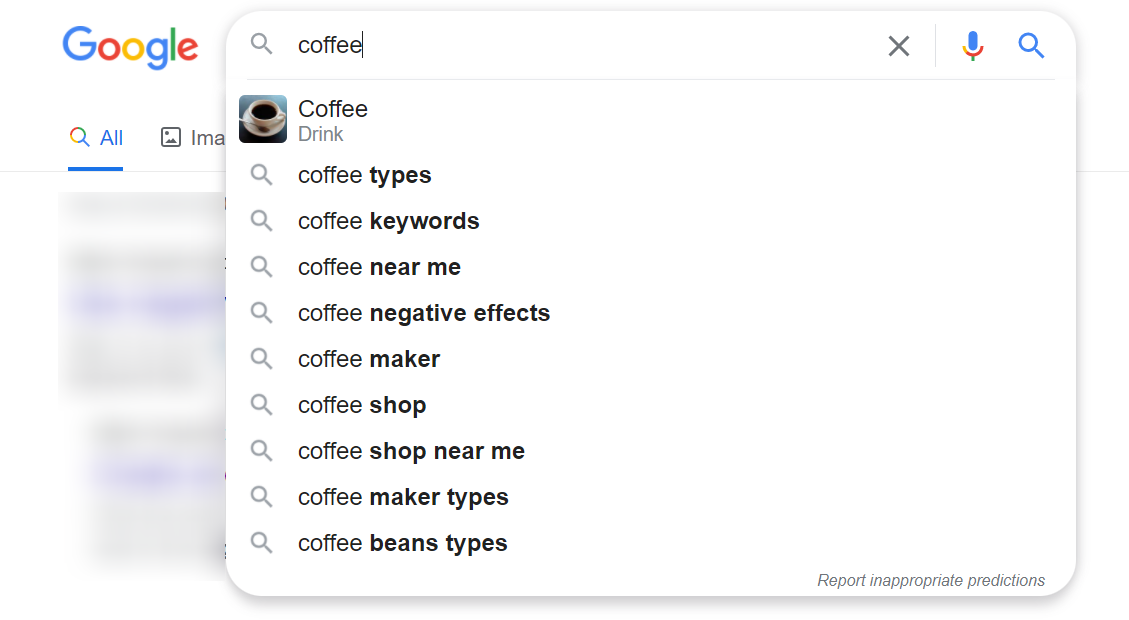A detailed Google search interface is shown with the keyword "coffee" typed into the search bar. The iconic Google logo, featuring its multicolored letters, is prominently displayed at the top of the screen. Underneath the search bar, a contextual suggestion box appears, partially obscuring the background results. The suggestions presented include "coffee drink," which is accompanied by a vibrant image of a steaming cup of coffee, and "coffee types." Other clickable autofill suggestions include "coffee keywords," "coffee near me," "coffee negative effects," "coffee maker," "coffee shop," "coffee shop near me," "coffee maker types," and "coffee beans types," each associated with a small magnifying glass icon. The background is intentionally blurred to emphasize the clarity and prominence of the search suggestions pop-up.